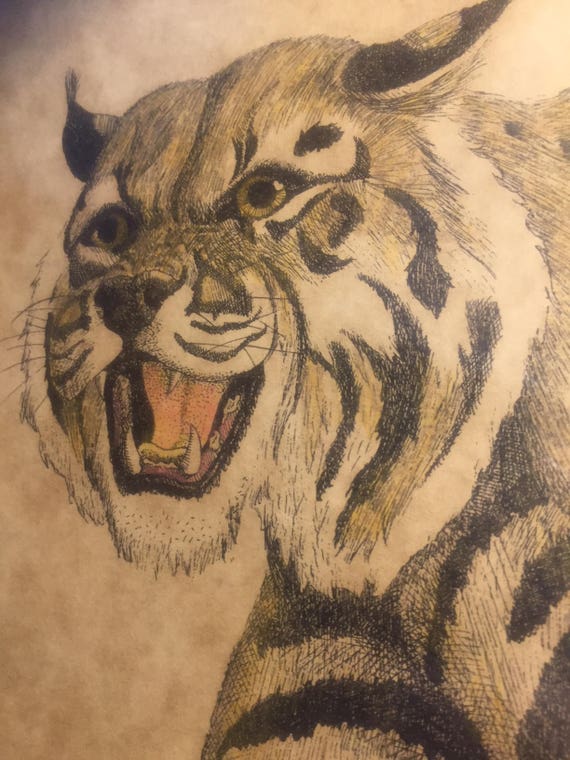The image features a detailed tattoo of a snarling tiger, showcasing impressive artistry. The tiger’s mouth is open, revealing sharp upper and lower canines and a pink tongue. The facial expression is fierce, with wide open eyes that have yellow irises and black pupils, and a snarled nose, contributing to its menacing look. The tiger's fur is an intricate blend of white, brown, black, and touches of golden hues, with black stripes seamlessly incorporated. A distinctive white ring of fur surrounds its chin and the outer edge of its neck. The ears, colored black with faint brown spots, are pricked forward, enhancing its alert and predatory demeanor. The background appears to be the tattooed individual’s white skin. Though the artwork is contemporary, it is detailed and vintage-inspired, reminiscent of Jean Murray's style. The faded coloring of grays, blacks, and beige also gives it an aged, classic look. Despite the lack of a visible signature, the tattoo's intricate details are compelling and memorable.